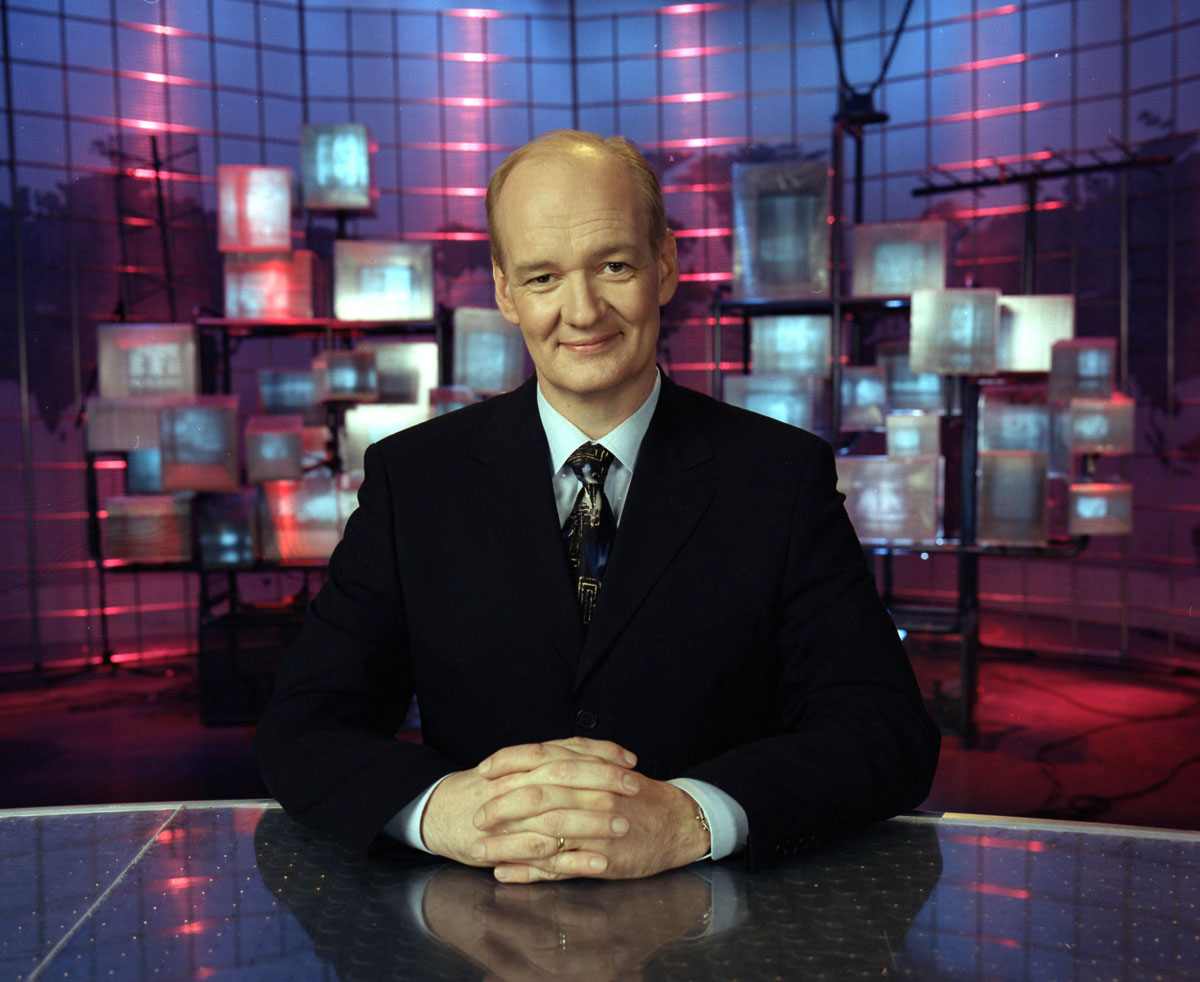This is a detailed photograph of Colin Mochrie seated at a sophisticated round table with gold trim and a dark, reflective glass top, which has intricate decorations embedded just beneath the surface. He has his hands folded in front of him and his head slightly tilted, displaying a neutral smirk. Colin is balding and has short-cropped hair. He is dressed in a dark suit jacket paired with a light blue or possibly white shirt and a dark blue tie. He also sports a wedding ring and a partially hidden watch under his shirt cuff. In the background, there is a set design comprising a series of transparent square panels, illuminated with a red light, giving an impression of a curved, modern space. The overall scene suggests a studio setting, potentially for a talk show or similar production.